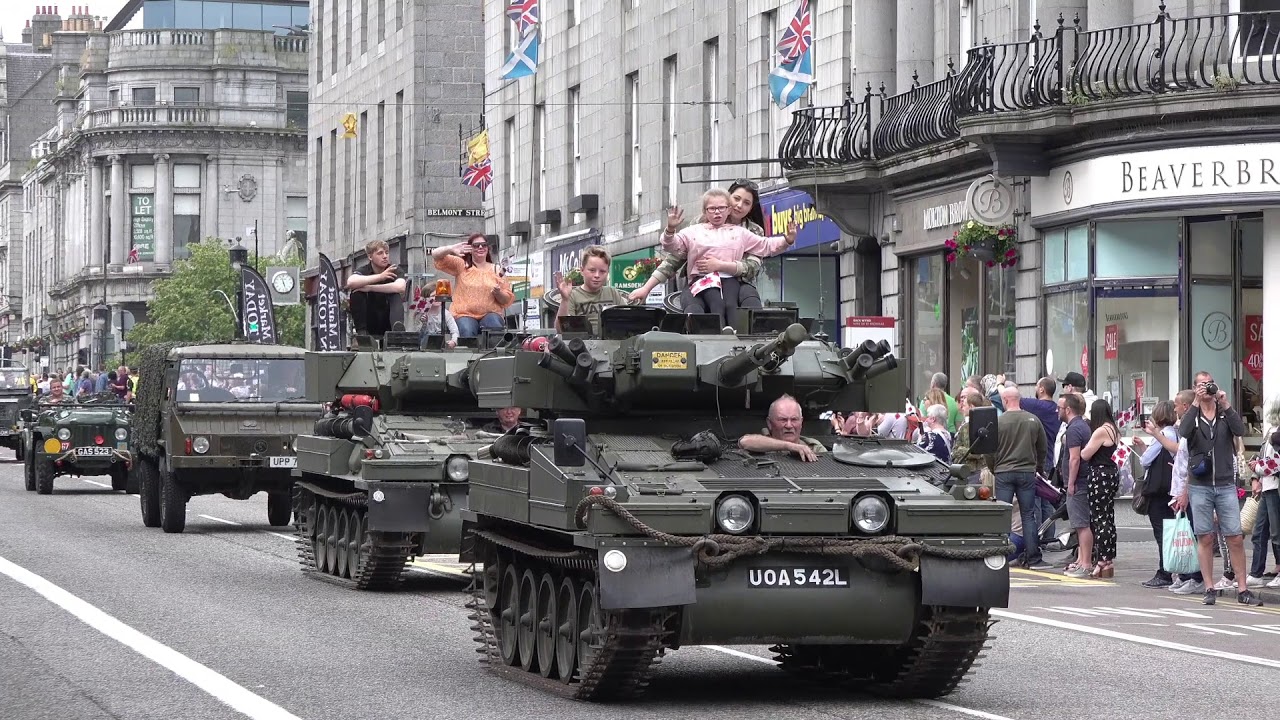This landscape-oriented, color photograph captures a vibrant street scene during a military parade in what appears to be a prominent city in Scotland, likely either Glasgow or Edinburgh. The streets are lined with onlookers, many of whom are eagerly snapping photos of the procession. Among them, families and children are excitedly waving from the sidewalks. The parade itself features several military vehicles, including two tanks and other military-style trucks and jeeps. The tanks are not the least bit intimidating due to their friendly passengers, which include children, an older man, a young woman, a mother, and a teenage son. The participants on these tanks appear to be family members of veterans, dressed in civilian clothes and radiating joy. The backdrop consists of classic, old-looking gray buildings adorned with various flags, notably the British Union Jack and the Scottish national flag. A nearby building emblazoned with the word "Beaver" also features a balcony, contributing to the charming atmosphere of this historic city's celebration.